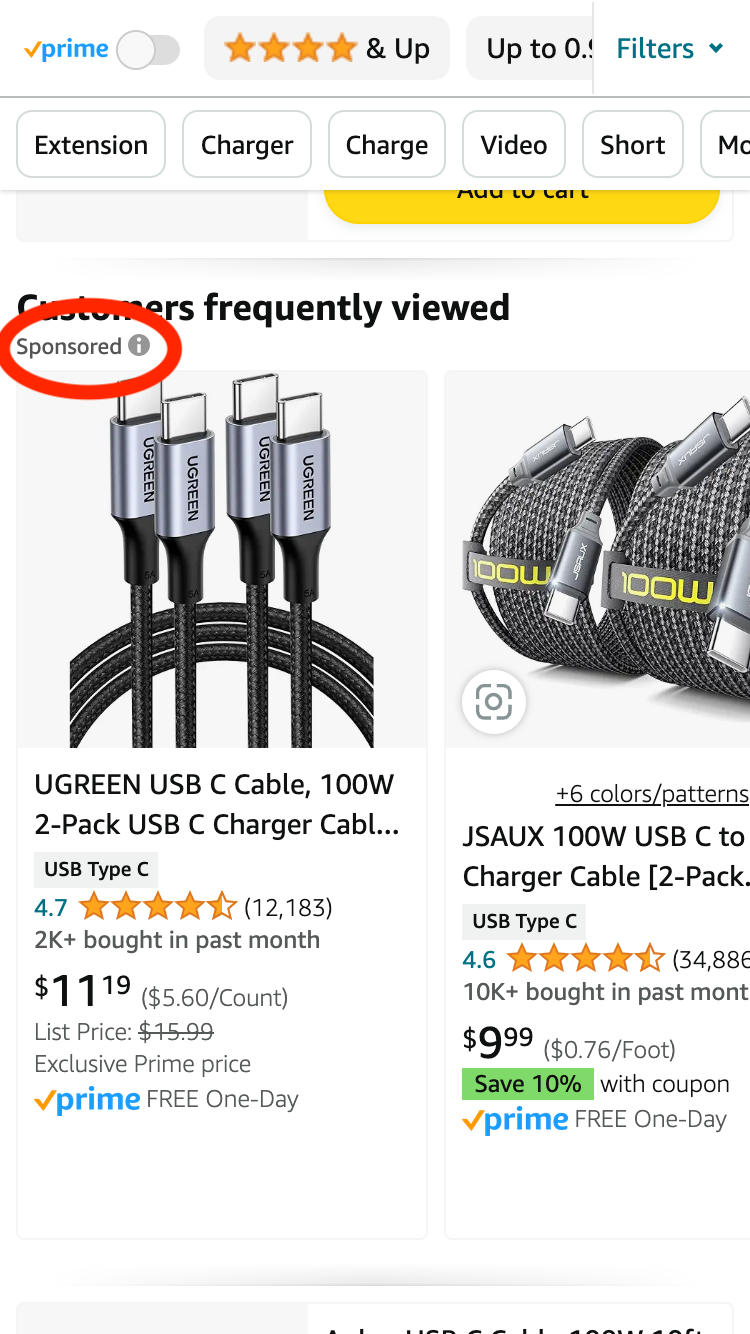The screenshot features a white background and predominantly displays a product listing with an emphasis on a USB Type-C charging cable set. At the top, there are toggle bars for "Prime" that are switched off, and a filter button highlighted in blue. The rating filter is set to "5 stars & Up." 

Midway down, a section labeled "Customers frequently viewed" is visible, followed by a "Sponsored" label circled in red, with a gray circle featuring a white "i" symbol inside it. 

The highlighted product is a "UGREEN USB C Cable, 100W, 2-Pack USB C Charger Cable." It is rated 4.7 stars out of 5 based on 12,183 reviews. The current price is $11.19, discounted from the original list price of $15.99. Notably, it includes the "Exclusive Prime Price" and offers "Prime Free One-Day Shipping."

Additionally, there is a listing for another product from JSAUX, labeled as "JSAUX 100W USB C to USB C Charger Cable (2-Pack)," which has a 4.6-star rating from 34,886 reviews. This product is priced at $9.99.